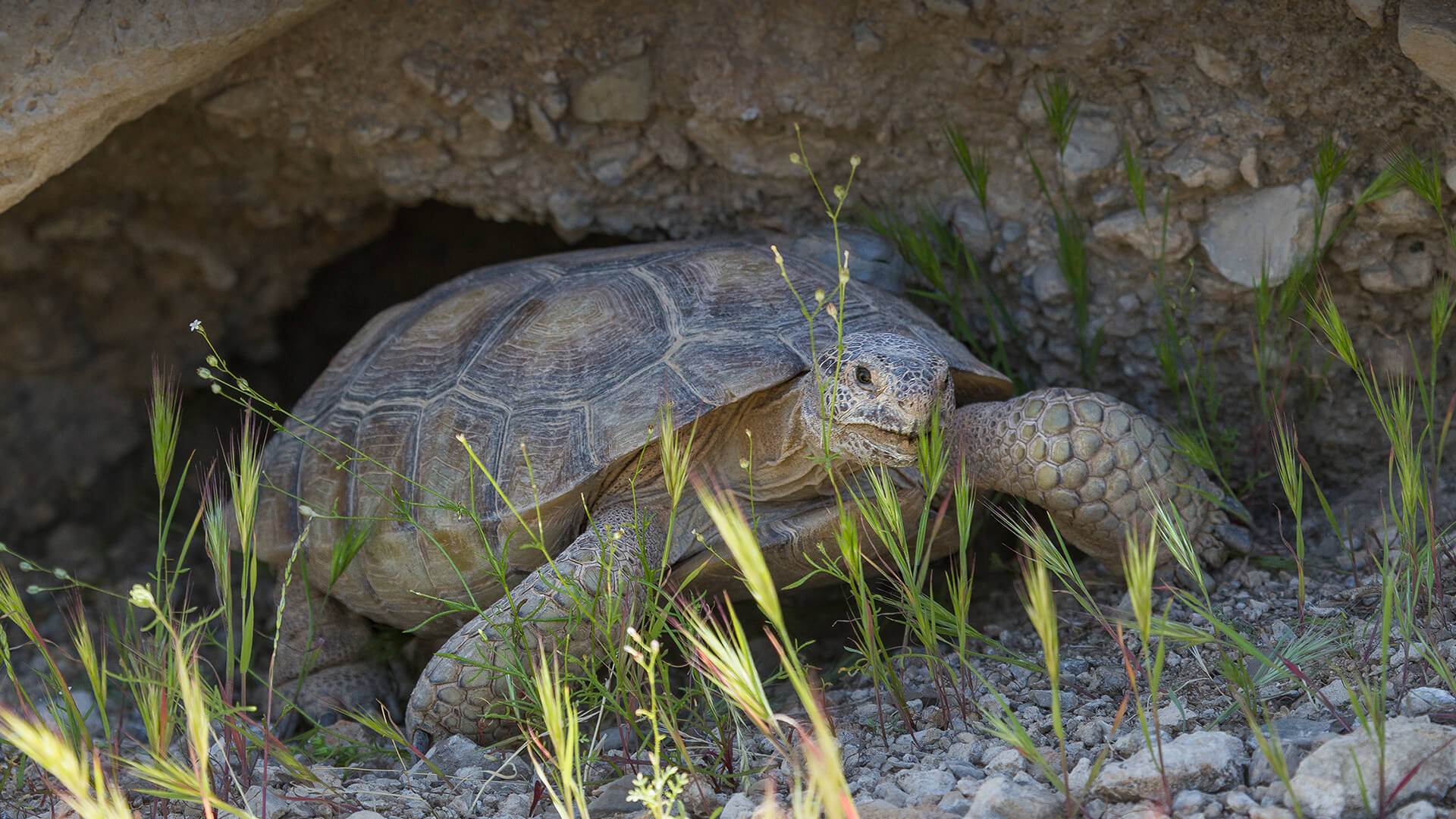In this detailed outdoor photo, an old, mature land turtle is depicted emerging from a rocky, cave-like opening. The scene suggests a warm, sunny environment as the turtle navigates a terrain covered in pebbles and stones interspersed with small sprouts of green foliage. The turtle, whose coloration includes shades of gray, beige, and brown, is positioned with one scaly leg in front of the other, indicating motion. Its heavy, segmented shell reveals intricate patterns, while the turtle's head, featuring small black eyes and an open mouth, appears to be directed towards the camera, possibly nibbling on the grass blades nearby. The cave-like structure curves around the turtle, with broken rock formations framing the scene and giving the impression of a natural, rugged habitat.